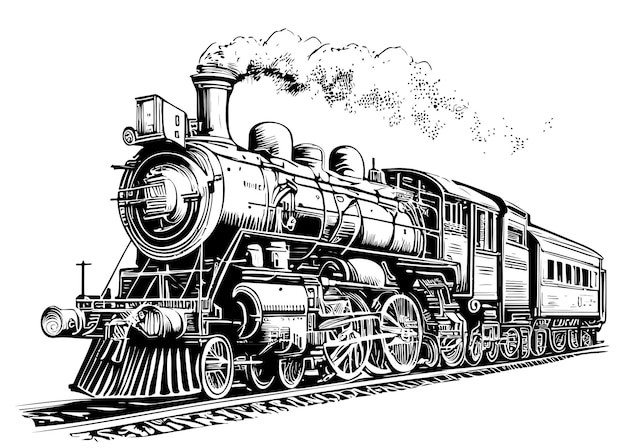The image depicts a black-and-white digital sketch of a historic steam train, traveling along a railroad track that moves diagonally from the bottom left to the middle right of the frame. The background is entirely white, focusing all attention on the intricately detailed train. The locomotive, emitting thick clouds of steam that gradually dissipate into black dots towards the rear, captures the eye with its bulky structure, reminiscent of older, pollution-heavy trains. The train appears to consist of a front engine and three carriages – a small one directly following the engine and a longer one at the end. The numerous wheels under the carriages emphasize its hefty build, reinforcing the historic feel of the illustration.